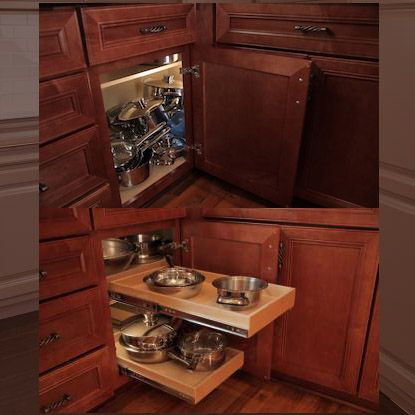Inside a kitchen with red-brown cabinets featuring bronze handles and a matching hardwood floor, a before-and-after transformation is showcased in two images. The top image reveals an open lower kitchen cabinet teeming with a disorganized mess of pots and pans, crowded and piled haphazardly. The cabinet interior, illuminated by a light, highlights the chaotic state within. In contrast, the bottom image presents the same cabinet, now fitted with two light wooden, pull-out drawers, enhancing the functionality and organization. These drawers neatly cradle the once scattered pots and pans, illustrating a practical solution that turns a cluttered cabinet into an orderly, efficient storage space.